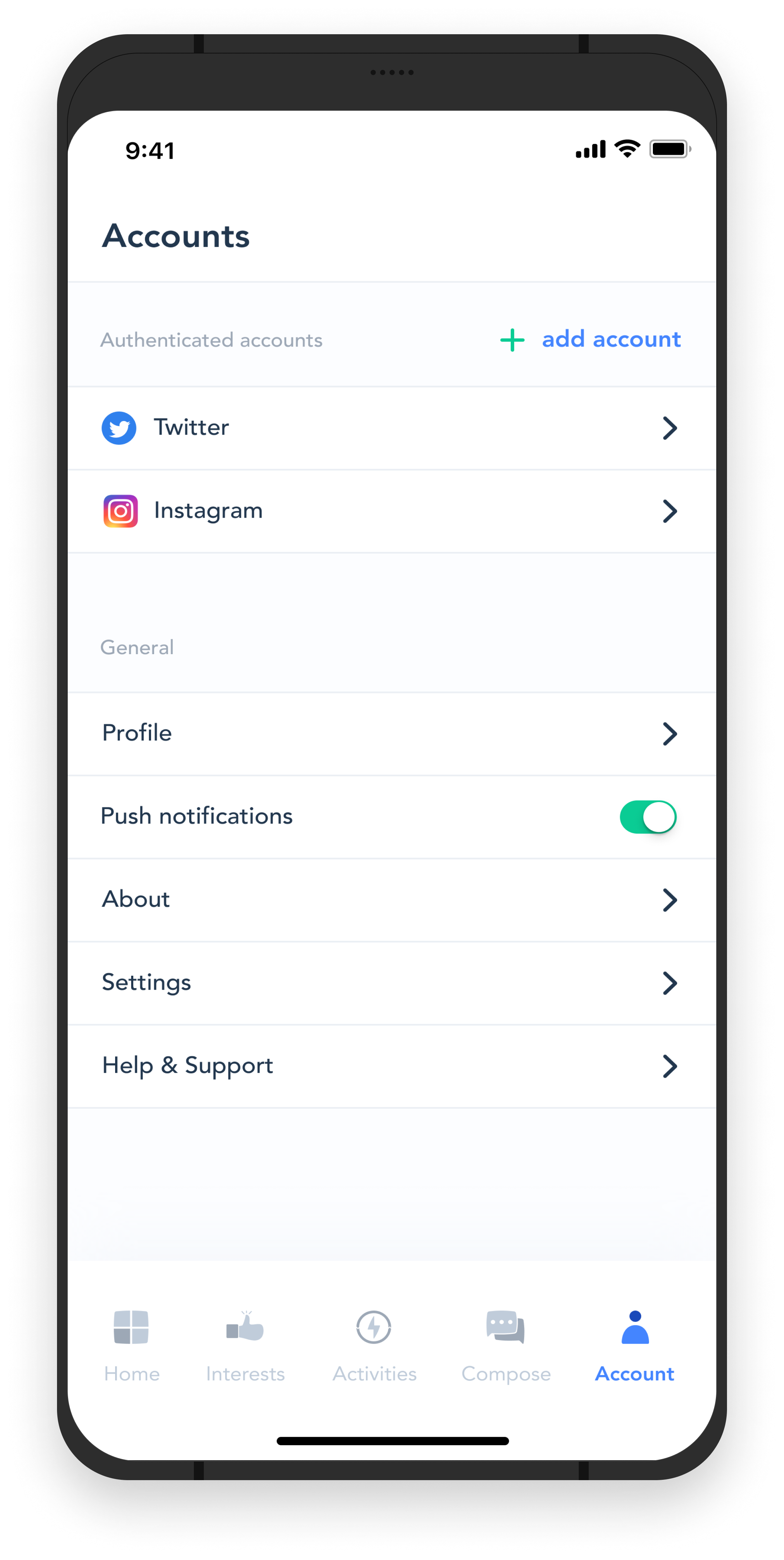This image is a detailed graphic of a smartphone screen, featuring a black bezel surrounding a simulated display. The screen shows a white status bar at the top displaying the time as 9:41, along with icons indicating full Wi-Fi strength, full mobile signal, and a full battery, all in black.

Below the status bar, the word "Accounts" is prominently displayed in black font. Further down, in a light blue rectangular box, the phrase "Authenticated Accounts" appears in gray font, accompanied by a blue-font "+ Add Account" option.

The image then features two white rectangular sections labeled "Twitter" and "Instagram," each accompanied by their respective logos and small right-pointing arrows at the end of these sections.

Further down, there is a section labeled "General" in gray font. Sub-sections include:
- "Profile" in a white rectangle
- "Push Notifications" with a toggle switch that is turned on
- "About," "Settings," and "Help and Support," each in white rectangles with right-pointing arrows indicating clickable options for expanding the menu.

At the very bottom of the screen, there are five icons corresponding to different navigation options: Home, Interests, Activities, Compose, and Account.